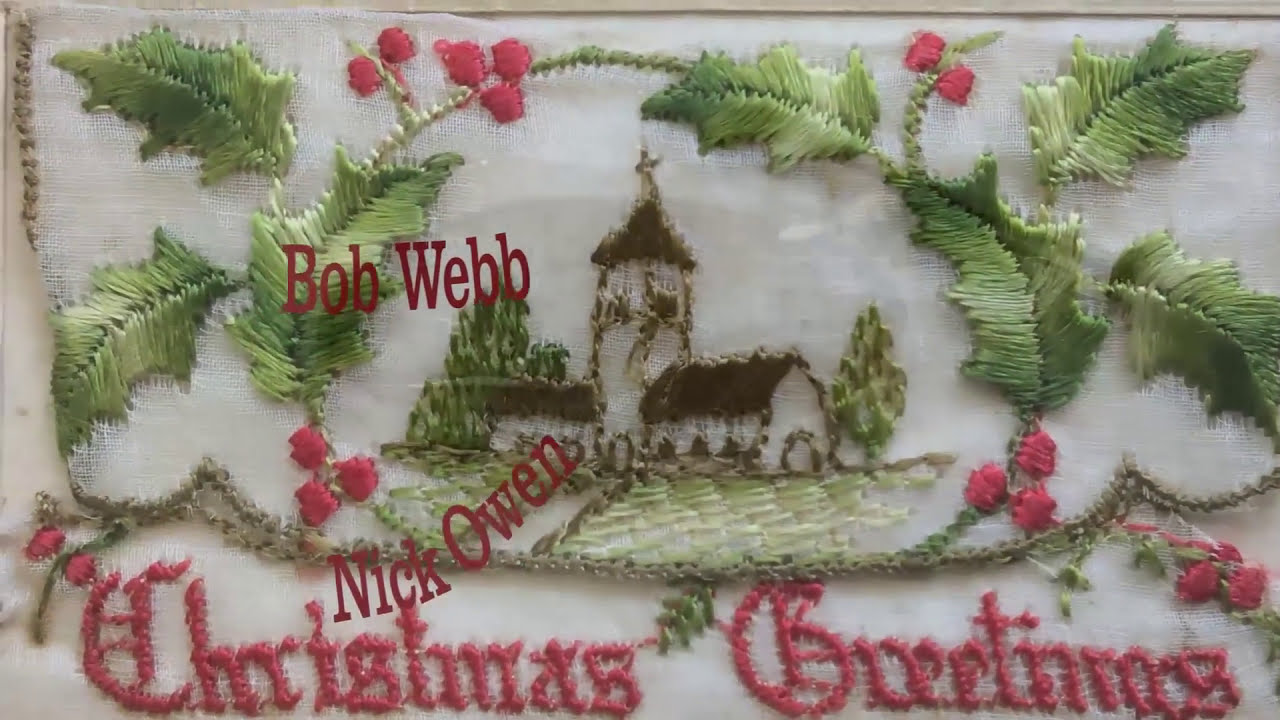This horizontal rectangular photograph displays an intricately decorated Christmas textile piece. The white backdrop serves as a canvas for the detailed knitted or quilted fabric. The textile features vibrant green leaves and festive red berries, reminiscent of holly, positioned along the upper left and right sides. Central to the design is the outline of a house, or possibly a church, with a prominent brown top on its tower and a smaller building beside it, flanked by green trees.

A green border frames this piece of cloth, adding coherence to the Christmas theme. At the bottom, the words "Christmas Greetings" are stitched in traditional red thread, lending a warm, festive message. Superimposed in red font on the photograph, the names "Bob Webb" and "Nick Owen" appear—Bob Webb's name at the top left and Nick Owen's name diagonally at the bottom left, giving a personalized touch to the image. The fabric's criss-crossed threads are visible, adding to the authenticity and handcrafted feel of this charming holiday decoration.